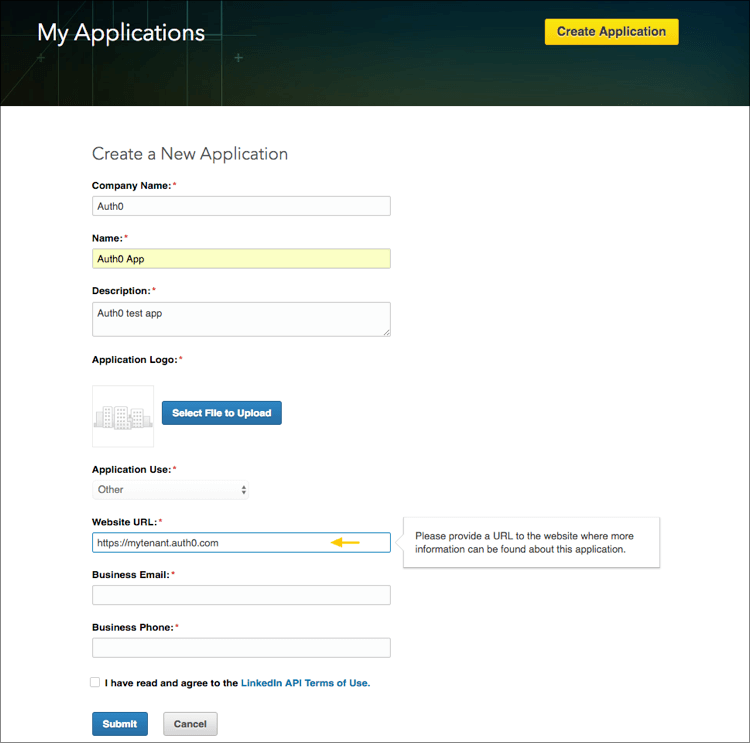This screenshot appears to be from a web application, likely an admin interface for Auth0. The design showcases a clean and organized layout with functional elements.

At the top, there's a black horizontal navigation bar. On the left side of the bar, in white text, it reads "My Applications". On the right side, there's a prominent yellow button labeled "Create Application" in black text.

Below the navigation bar, the main content area predominantly features black text on a white background, maintaining clarity and readability. 

Key elements include:
1. **Title**: "Create a New Application"
2. **Fields**: 
   - **Company Name**: Appears to be Airbnb, based on partial visibility.
   - **Auth0 Application Name**: The text indicates it’s an Auth0, but the field name isn't clearly stated.
   - **Description**: A brief abstract of the application details.
   - **Logo**: A placeholder square logo depicting faint pencil-drawn skyscrapers.
   - **Upload Logo**: A blue button with white text labeled "Select File to Upload".
   - **Application URL**: Pre-filled with "https://mytenant.auth0.com", alongside a small yellow arrow.

On the right side of the form, a message bubble provides guidance: "Please provide the URL to the website where more information can be found about this application."

Additional fields are present for business contact details:
- **Business Email**: Currently empty.
- **Business Phone**: Currently empty.

A mandatory agreement section is also present, requiring users to tick a box stating "I have read and agreed to the LinkedIn API terms of use", with the terms linked in blue text. This box is unticked.

At the bottom, two action buttons are available:
- **Submit**: Blue with white text.
- **Cancel**: Gray with black text.

Overall, the form is structured to gather essential information and facilitate the creation of a new application within the Auth0 platform.